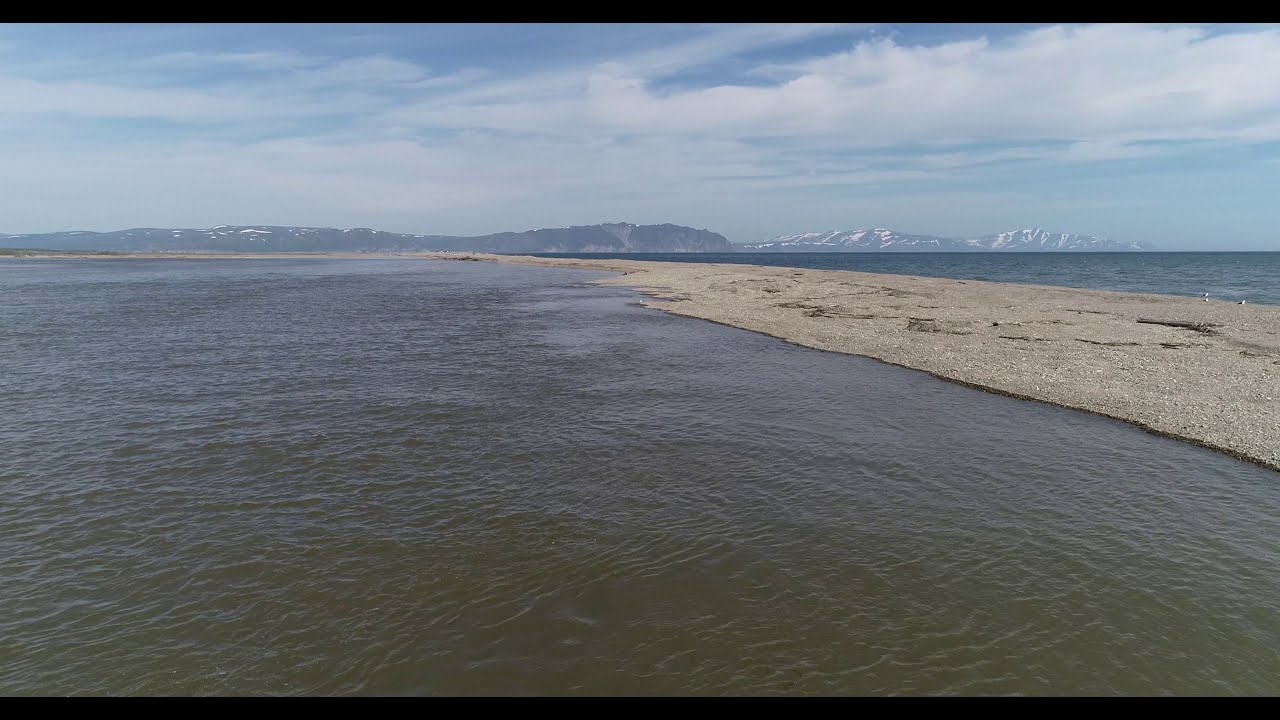In this detailed photograph taken from a slightly elevated viewpoint, we observe a tranquil scene dominated by a sprawling, blue-colored body of water that encompasses most of the image. This expanse of water, which appears to be a sea or lake, is divided by a rocky, beige-brown stretch of ground forming an L-shape that extends from the right side and curves towards the center, giving the impression of a natural pathway cutting through the water. On the far left, the water takes on a slightly brownish hue.

Beyond this rocky shoreline, the scene unfolds into a picturesque vista of towering mountains and hills in the distance. To the left, a dark-hued mountain contrasts sharply with another peak on the right, which is capped in white, indicative of snow. Further adding to the serene ambiance, the sky above is a brilliant blue dotted with soft, white clouds stretching towards the upper right of the photograph, creating a sense of depth and vastness. The entire image is a horizontal rectangle, capturing the quiet beauty of a daytime landscape at the water's edge. The color palette includes shades of blue, white, brown, beige, gray, and black, highlighting the natural elements present in the scene.